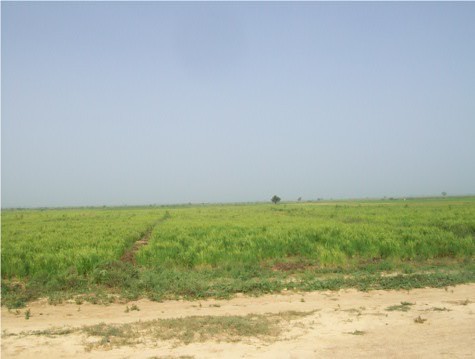This is a photograph of a flat, green marsh field with a worn dirt path, possibly a dirt road, running through it. The field is covered in medium-tall vegetation that could be crops, with patches of grass interspersed with hard-packed, light brown to reddish dirt. In the far distance, there's a solitary tree and possibly a couple more indistinct trees further out. The sky occupies half of the image, displaying a hazy, pale blue with some possible misty clouds. The scene is entirely outdoors with no buildings, people, or textual details, and the photograph itself is quite small, approximately three by three inches.